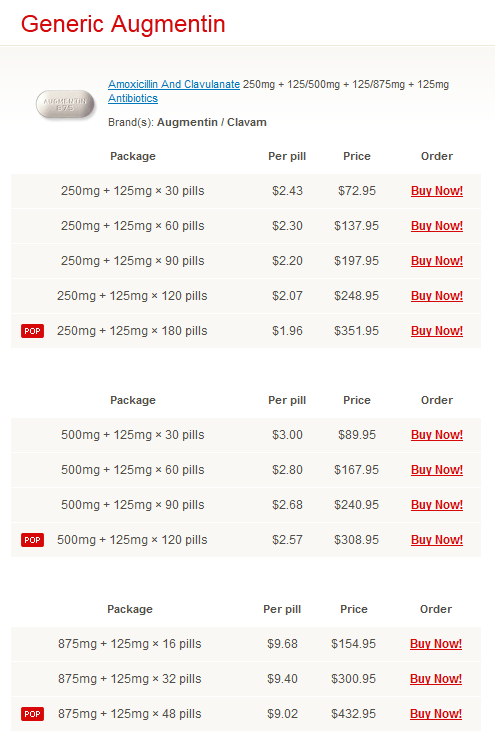The image features a detailed overview of a pharmaceutical drug, specifically a generic version of Augmentin. At the top, prominently displayed in red text, is the name "Generic Augmentin." Below this, an image of an oval-shaped, white Augmentin pill is shown, marked with the number "875." 

To the right of the pill image, the words "Amoxicillin and Clavulanate Antibiotics" are highlighted in blue, suggesting a clickable hyperlink. The text further mentions associated brands, "Augmentin/Clavum."

Various dosage packages are listed with their corresponding prices and quantities:
- **250mg + 125mg:** Available in packs of 30, 60, 90, 120, and 180 pills. The price per pill decreases with larger quantities, starting at $2.43 for 30 pills, and reducing to $1.96 for 180 pills.
- **500mg + 125mg:** Available in packs of 30, 60, 90, and 120 pills. The price per pill starts at $3 for 30 pills and decreases to $2.57 for 120 pills.
- **875mg:** Available in packs of 16, 32, and 48 pills. The price per pill ranges from $9.68 for 16 pills to $9.02 for 48 pills.

On the right-hand side of the image, there's an option to order the medication via a "Buy Now" hyperlink. The caption provides a comprehensive account of the product offerings, emphasizing the cost-effectiveness of purchasing in larger quantities.